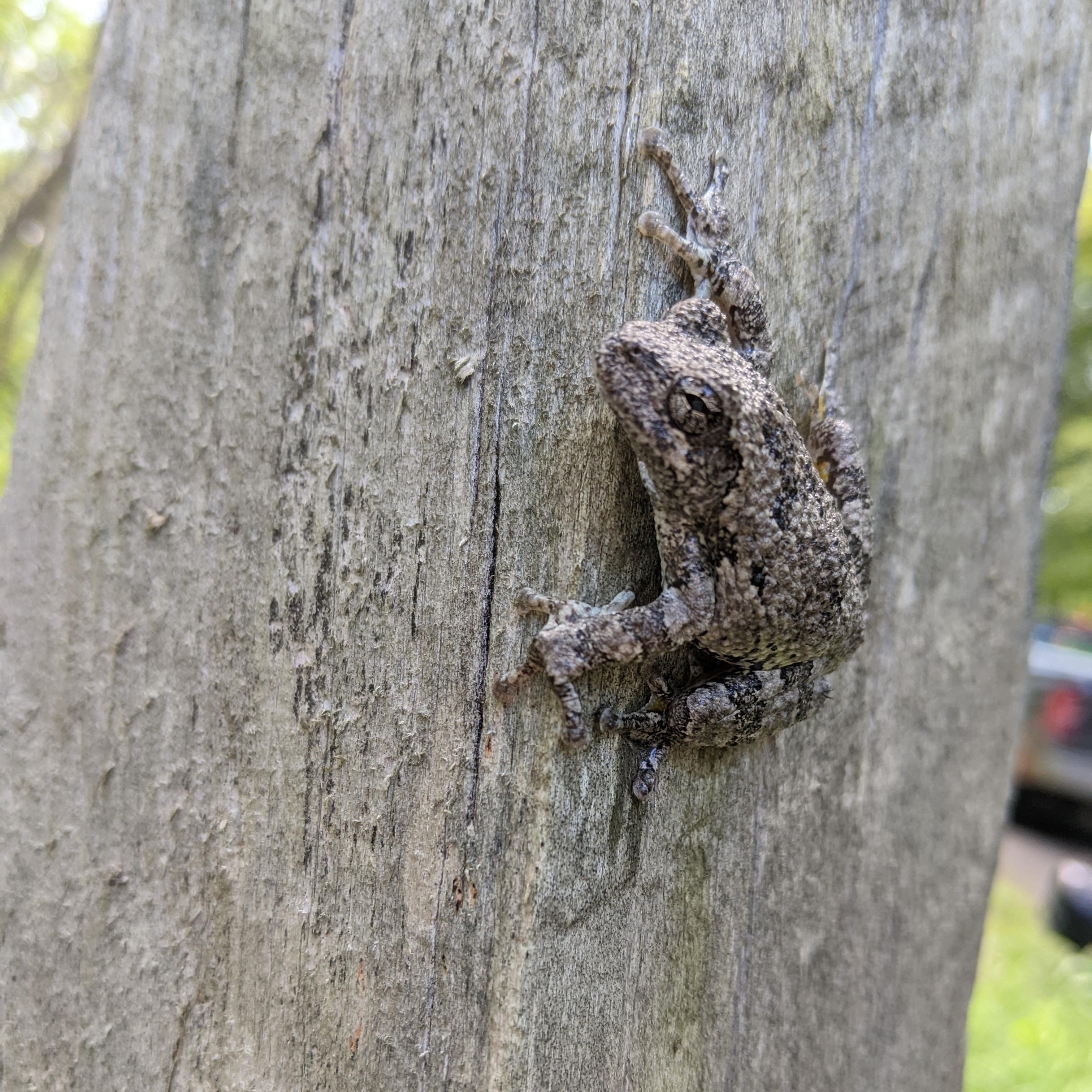This is a detailed photograph captured in daytime, focusing closely on a medium-sized tree trunk that appears to lack bark, revealing a light gray, exposed wood with darker vertical grain. The center of attention is a frog or toad clinging to the trunk. The amphibian’s skin features shades of gray, brown, and cream with black pebbled patterns that blend seamlessly with the tree, providing an impressive camouflage. The frog's eyes are mostly closed with just a hint of black slit pupils visible. Only the left side of its body can be seen clearly, with its right front leg positioned above the left as it clings to the trunk. The background is blurred, showing hints of green grass, blurry branches, and a distant car park, which accentuates the sharp focus on the intricately camouflaged frog.